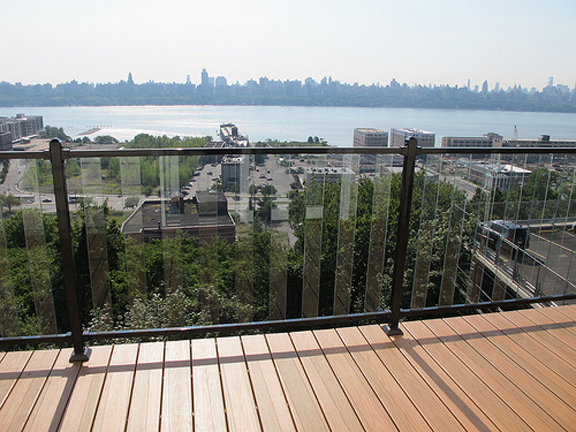The image captures an urban cityscape viewed from a high-rise building's wooden porch with slatted brown deck boards. The black railing, adorned with vertical glass panels, lines the edge of the porch. Below, an expanse of green trees stretches over roads bustling with traffic and parking lots, including one atop a nearby building. The midground reveals a vast, blue body of water, seemingly nestled between the foreground's greenery and the background cityscape. The distant horizon is dotted with numerous tall buildings, both residential and industrial, silhouetted against a bright daytime sky. Shadows cast a dark gray hue horizontally and vertically across the wooden deck, enhancing the image's depth and texture.